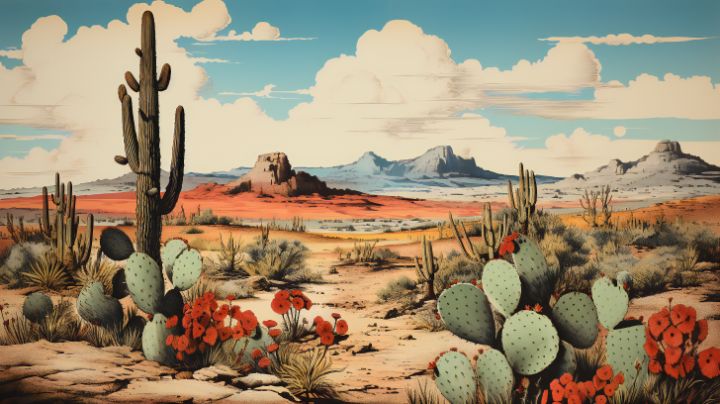This vintage painting portrays a vibrant desert landscape, reminiscent of Monument Valley in Arizona, often seen on old postcards or cigar boxes. The foreground showcases an array of detailed flora, including prickly pear cactuses, characterized by their paddle-like, thorn-covered segments that occasionally bear red fruits. Scattered among these are striking red flowers and possibly some yucca plants. Towering over the scene are the iconic saguaro cacti, firmly standing with their large, upward-reaching arms, evoking the classic imagery of Westerns.

The arid terrain extends into the distance, gradually shifting from an orangish-brown to a lighter pink and tan hue. Far off, the landscape transforms into the majestic buttes and flat-topped mesas, sculpted by erosion, that define Monument Valley's rugged beauty. Above this expansive desert, the sky is a mix of blue and cloudy, adding depth and texture to the scene. This finely crafted illustration captures the essence of the southwestern desert, blending the unique vegetation and the dramatic geological formations into a timeless, picturesque vista.